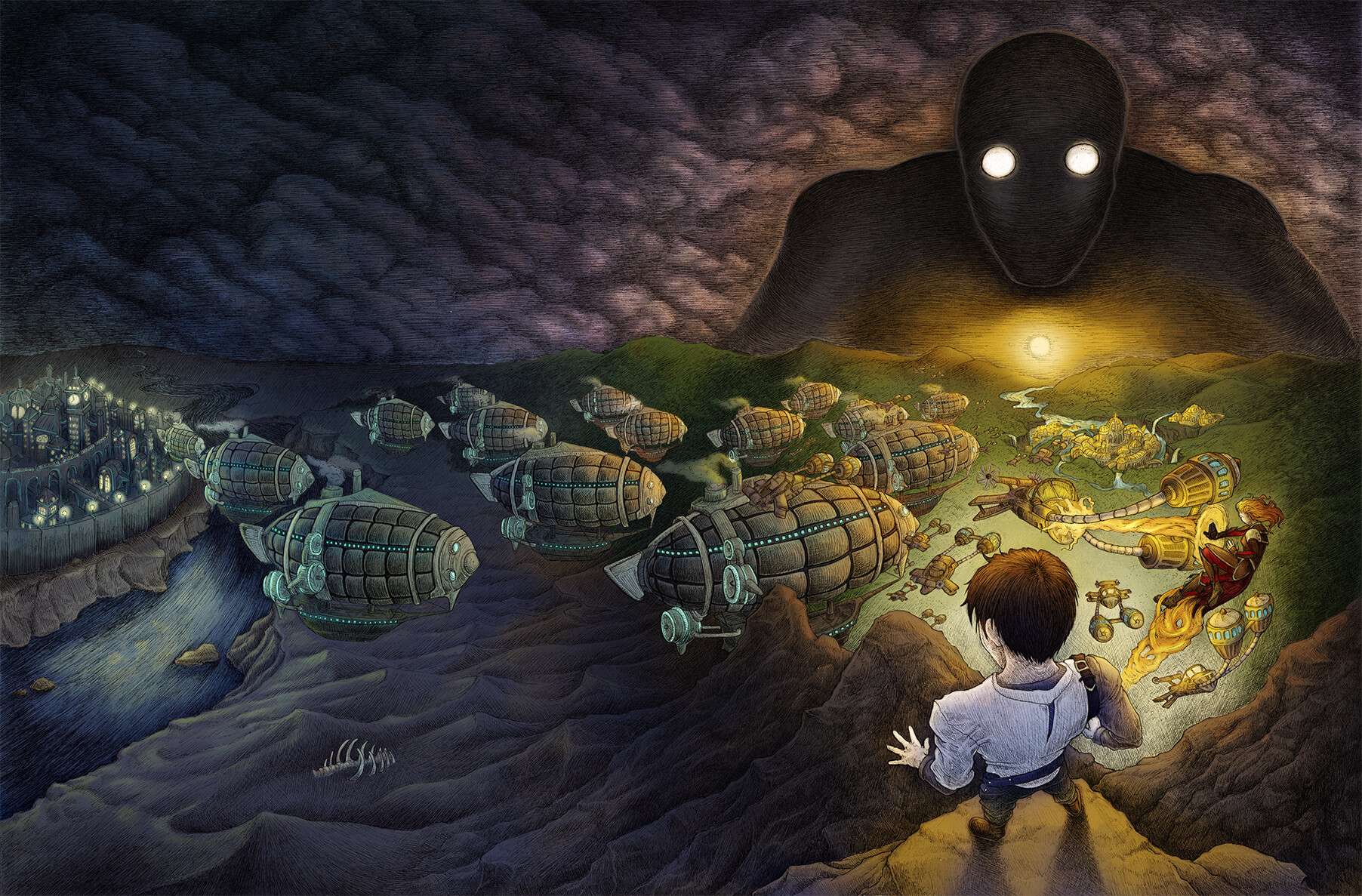In this animated, comic-style illustration, a young man with short brown hair and dressed in a white shirt stands on a rocky ledge, looking down at a dynamic underwater scene. Below him, the water transitions from blue on the left to green on the right, where numerous submarine-like vessels float, resembling hand grenades. To the left, a city with numerous bright lights is partially visible, suggesting a subterranean, possibly sea-based, civilization. The backdrop features a dark purple sky with light purple clouds, adding to the mysterious atmosphere. In the upper right-hand corner, a looming, monstrous silhouette with glowing white eyes watches over the unfolding events, hinting at an adventure or impending conflict. The composition and elements suggest the young man might be a central figure, possibly the hero of an action-packed storyline.